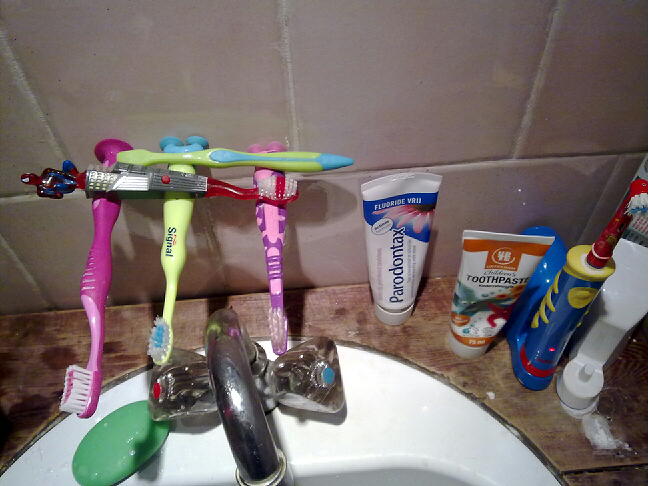This is a detailed color photograph taken inside a bathroom, specifically focusing on the area around the sink. The image showcases a white sink with wooden-looking countertops, backed by a tiled wall. The sink features two traditional faucet knobs marked with red and blue, evoking a nostalgic feel.

Attached to the tile wall above the sink are three toothbrushes: one is pink, another is green, and a smaller pink one, all held in place by suction cups. Horizontally resting atop these suction-cupped toothbrushes are two more: a Spider-Man-themed toothbrush and another small green one. On the countertop below, various dental hygiene items are visible, including two bottles of toothpaste, one labeled "Peridontics" and another simply marked as "toothpaste." Additionally, a blue electric toothbrush and a bar of green hand soap are present.

The countertop shows some white powder residue in the bottom right corner, adding a lived-in touch to the scene. The arrangement of toothbrushes and other items gives an impression of a busy and practical family bathroom setup.